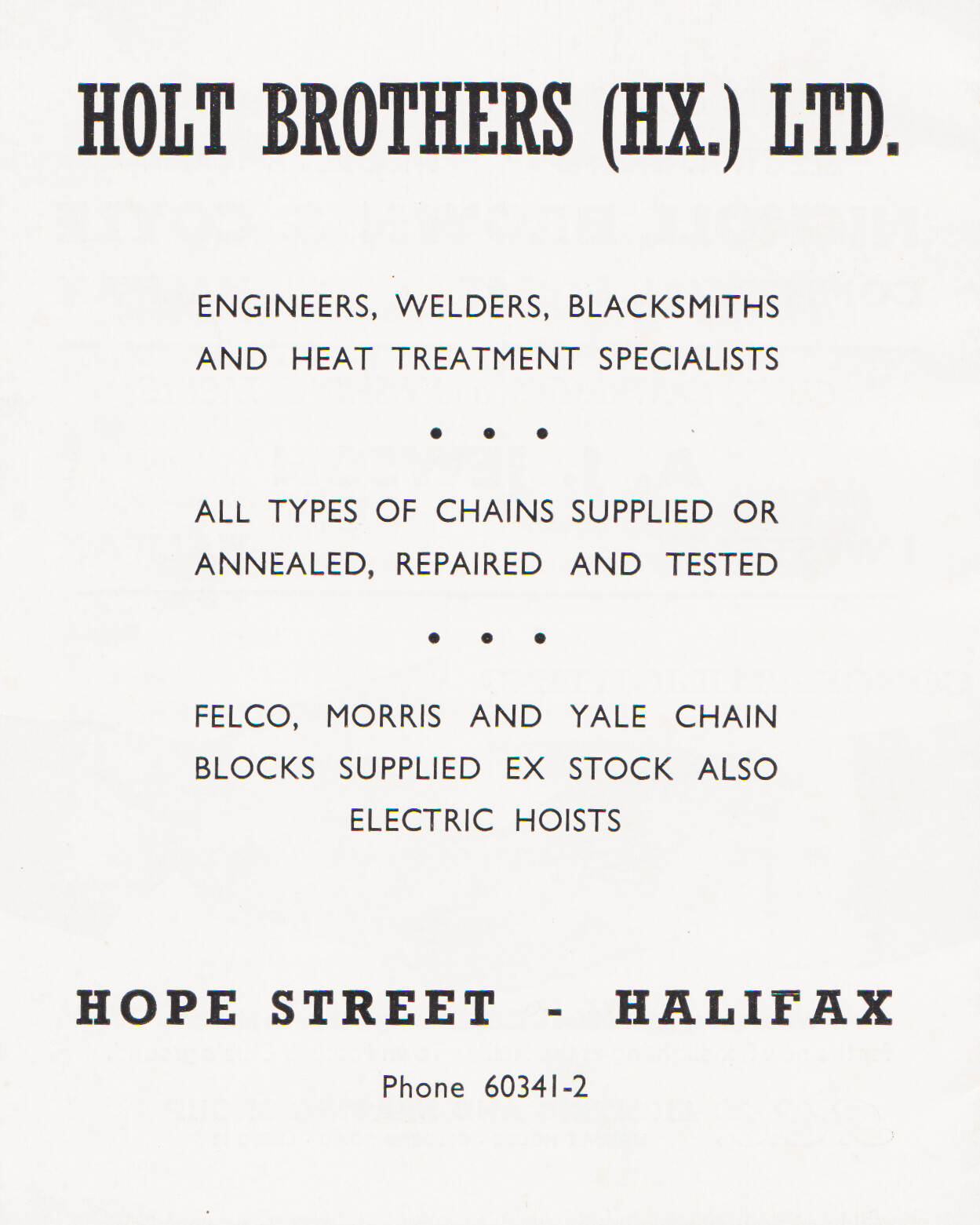The image displays a text-based advertisement on an off-white or light gray background, featuring bold, centered, black text. At the top, in larger, all-capital letters, it reads "Holt Brothers (HXLTD)." Just below, it mentions "ENGINEERS, WELDERS, BLACKSMITHS, AND HEAT TREATMENT SPECIALISTS." This is followed by a three-dot horizontal separator. The ad continues with "ALL TYPES OF CHAINS SUPPLIED OR ANNEALED, REPAIRED, AND TESTED," then another three-dot separator. It lists brands with "FELCO, MORRIS, AND YALE CHAIN BLOCKS SUPPLIED. X-STOCK, ALSO ELECTRIC HOISTS." At the bottom, in bold black text, it states "HOPE STREET, HALIFAX," and underneath in smaller text, "Phone 60341-2," indicating it might be an older page.